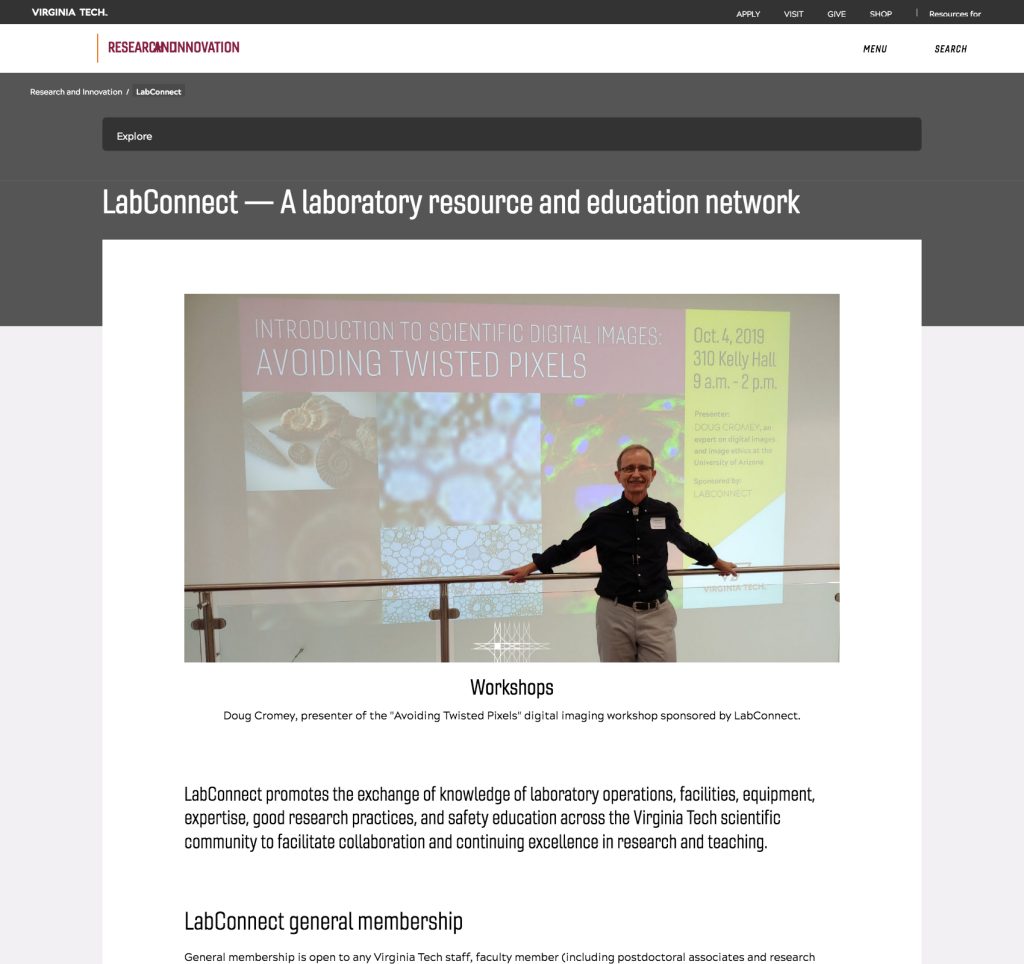At the top of the image, "Virginia Tech" is prominently displayed. Below it, options such as "Apply," "Visit," "Give," "Shop," and "Resources for" are listed. A white rectangle with a red vertical line features the text "Research & Innovation," and a menu includes options like "Search," "Research and Innovation," and "LabConnect."

Beneath this, a dark gray bar with the word "Explore" appears. The main focus is on the "LabConnect – A Laboratory Resource and Education Network" section. This image promotes an "Introduction to Scientific Digital Images: Avoiding Twisted Pixels" workshop, held on October 4, 2019, from 9 a.m. to 2 p.m. at 310 Kelly Hall.

In the background, there are various images related to scientific research. The workshop, presented by Doug Cromier, is part of LabConnect's initiatives. LabConnect aims to foster the exchange of knowledge regarding laboratory operations, facilities, equipment, expertise, careers, practice, and education within Virginia Tech's scientific community to encourage collaboration and uphold excellence in research and teaching. The image also notes that general membership to LabConnect is open to any Virginia Tech staff.